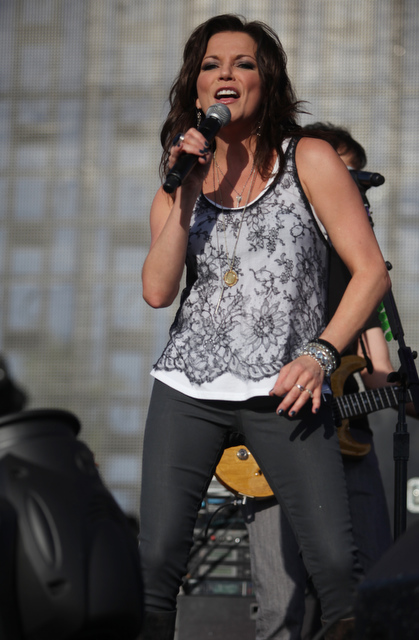In this color photograph, a woman who resembles Martina McBride is captured mid-performance on stage. She has long, straight, and slightly wavy dark brown hair and wears light red lipstick. She's dressed in tight grey pants and a black and white tank top with a grey floral pattern, layered over a white undershirt. In her right hand, she holds a black microphone close to her mouth, which reveals her top teeth as she sings. Her nails are painted black, and on her left wrist, she wears silver bracelets along with several silver rings scattered across both hands. Behind her, partially obscured, is a man playing a brown guitar with a microphone positioned near him. The backdrop features a grey, blurry plaid design in shades of brown and blue. In the bottom right corner of the image, a piece of black equipment is faintly visible.